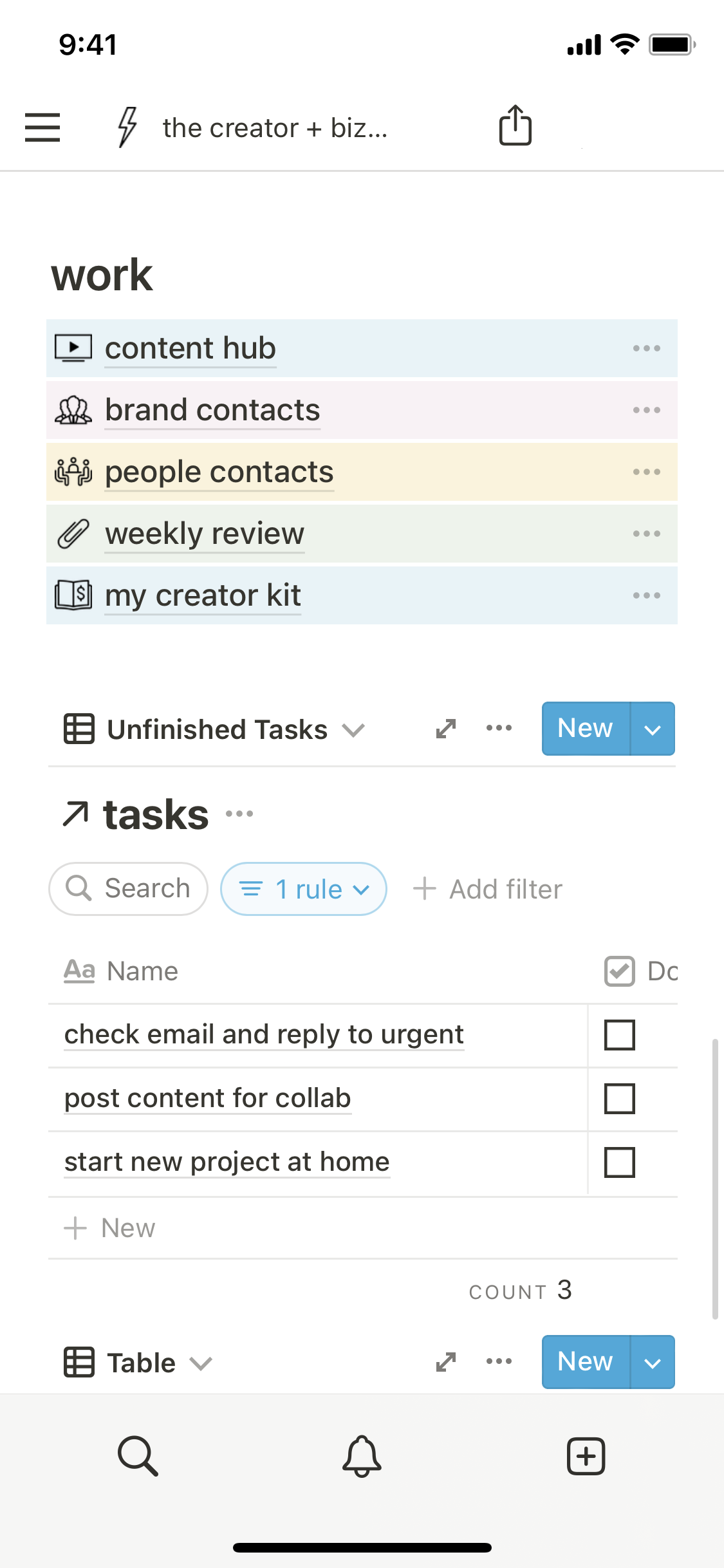This is a screenshot of a mobile productivity application interface. At the very top left corner, in bold black text, is the current time displayed as "9:41." The top right corner features the signal strength icon, Wi-Fi signal icon, and a fully charged battery indicator.

Below the status bar, on the left side, there is a hamburger menu icon (three horizontal lines stacked on top of each other). Next to it, moving from left to right, is a lightning bolt icon followed by text reading "Creator Plus Biz...", which is partially obscured. There’s also an icon for forwarding or transferring files, depicted as a box with an upward arrow emanating from the top.

Underneath this row, a bold black header reads "Work." Below this header are clickable options arranged in rows: "Content Hub," "Brand Contacts," "People Contacts," "Weekly Review," and "My Creator Kit."

The section titled "Unfinished Task" is next, featuring a blue "New" button on the right side for adding new tasks. Below this button is an unmarked checklist containing three items: "Check email and reply to urgent," "Post current content for collab," and "Start new project at home."

Overall, the interface appears to be designed for managing various tasks and projects efficiently, catering specifically to content creators.